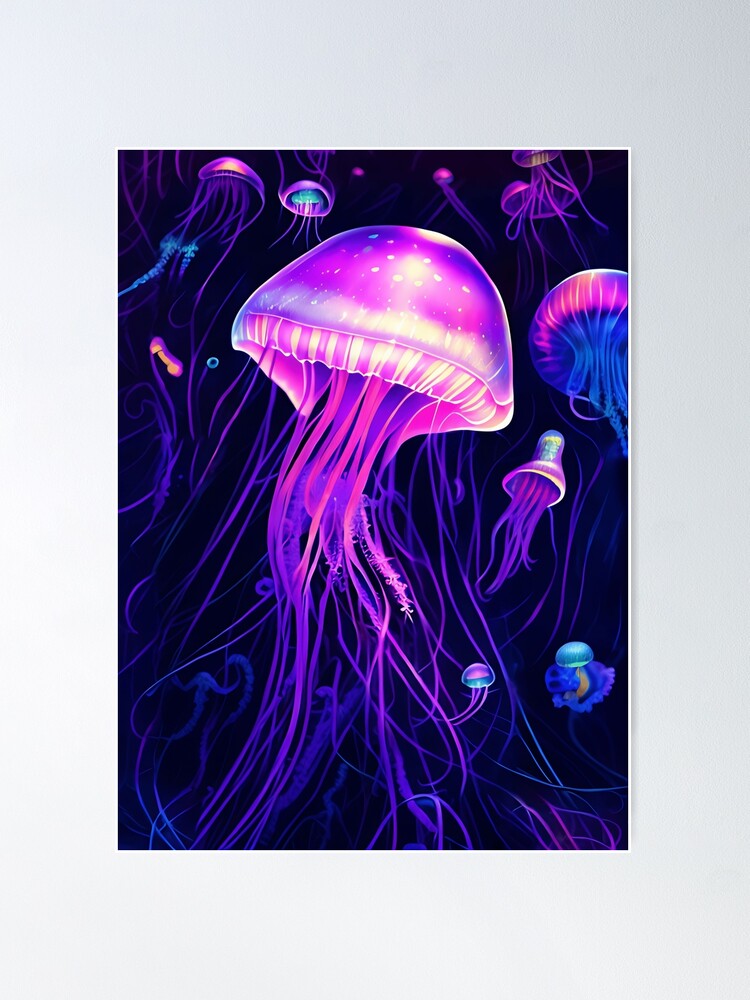In this vibrant animated digital illustration, a series of luminescent jellyfish float gracefully against a predominantly dark, almost black, background. At the forefront of the image, the largest and most prominent jellyfish displays a radiant gradient from dark purple to lighter purples, pinks, and whites, with tendrils transitioning from darker purples to pinkish hues, exuding a mesmerizing glow. Surrounding this central figure, several smaller jellyfish drift in the background, featuring caps of fluorescent pink and aqua, with tendrils in shades of blue and pink. These jellyfish effectively add depth and intrigue to the composition. The scene is punctuated by other mysterious geometrical objects, including a donut-shaped sphere and an enigmatic, skull-like figure in dark blue at the bottom right, adding a touch of eerie fascination to the otherwise ethereal underwater tableau.